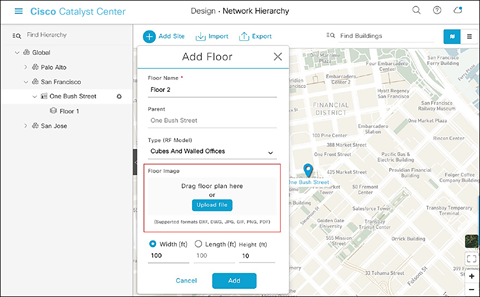Detailed Caption: 

This image, taken from a web page called Cisco Catalyst Center, features a prominently displayed teal icon and the site's name in teal text positioned in the upper left-hand corner. Adjacent to this, the phrase "Design Network Hierarchy" is written in black font. 

In the upper right-hand corner, three distinct icons can be seen: a magnifying glass, a question mark, and a cloud with a dot. 

Moving down the page, a left-hand sidebar displays a list of locations including "Find Hierarchy," "Global," "Palo Alto," "San Francisco," "1 Bush Street, Floor 1," and "San Jose." 

In the central area of the page, there's a series of buttons and options such as "Add Site," "Import and Export," and "Find Buildings." 

Additionally, there is a detailed map with a teal pin indicating the location of Bush Street. A pop-up overlay is also visible, displaying options to "Add Floor" with the input field pre-filled as "Floor 2." 

Further details include "Parent: 1 Bush Street," "Type: Cubes and Walled Offices," followed by a red rectangle containing the text "Floor Image, Drag Floor Plan Here, or Upload File," along with buttons for "Upload File" and "Add."